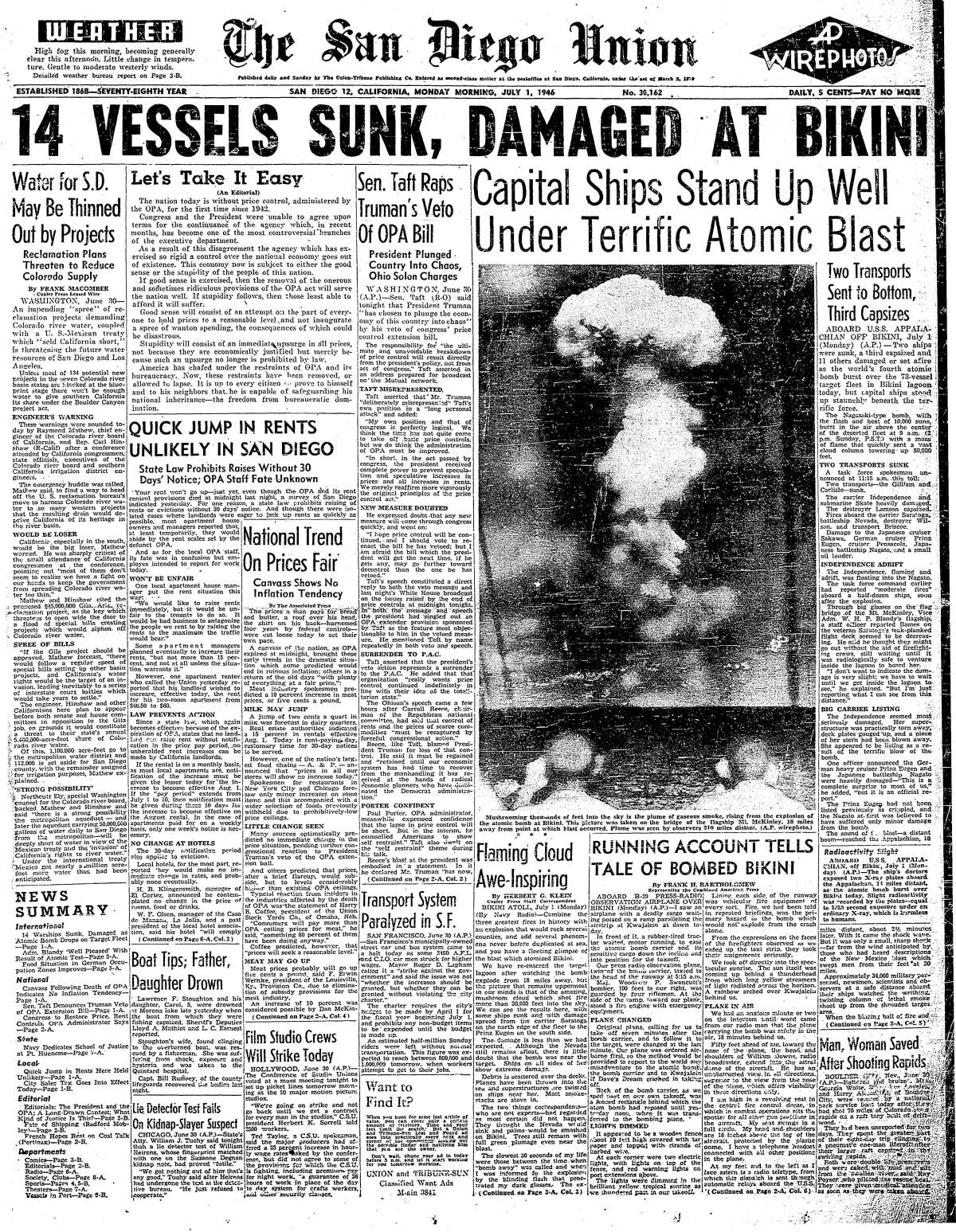This image captures a high-quality scan of the front page of the San Diego Union dated Monday morning, July 1, 1946, in its 78th year of publication since its establishment in 1868. Priced at five cents, the paper features a prominent header indicating the inclusion of AP wire photos. Dominating the page is the headline, "14 Vessels Sunk, Damaged at Bikini," with sub-headlines elaborating, "Capital Ships Stand Up Well Under Terrific Atomic Blast" and "Two Transports Sent to Bottom, Third Capsizes." Below this, there is a grainy black-and-white photo depicting two individuals wearing ear protectors, gazing at a massive mushroom cloud over water, captioned as, "Flaming Cloud, Awe-inspiring." Numerous smaller articles and headlines populate the page, with topics ranging from local concerns such as "Water for SD may be thinned out for projects" and "Quick jump in rents unlikely in San Diego" to broader issues including "Sen Tuff reps Truman's veto of OPA bill" and "National trend of prices fair." The comprehensive coverage reflects the era's pressing issues and the profound impact of atomic testing at Bikini Atoll.